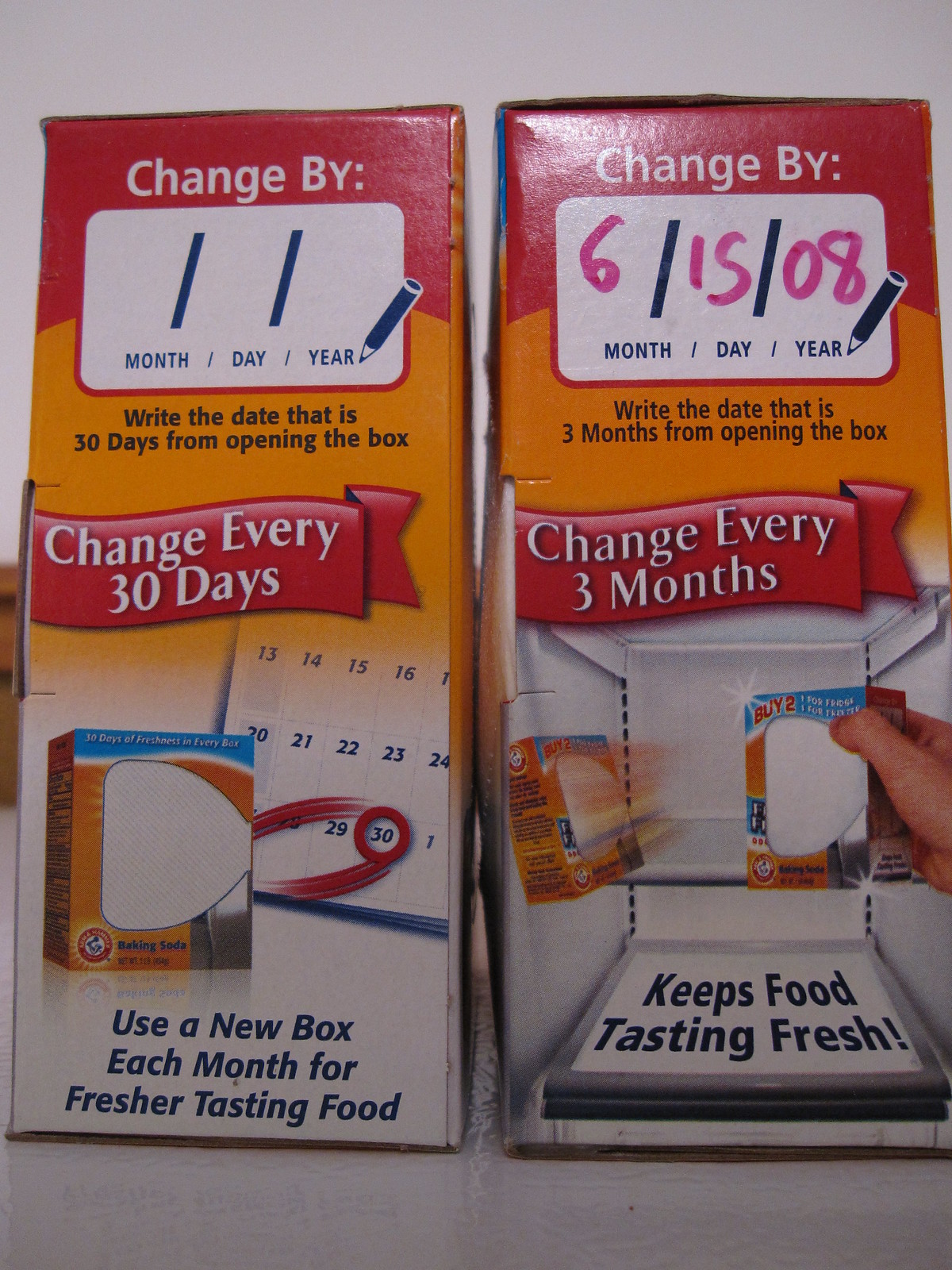This photograph depicts two side-by-side boxes of Arm & Hammer baking soda set against a gray, likely marble or granite, background. Both boxes feature a red top border, a yellow section underneath, and white on the bottom, resembling the interior of a refrigerator. 

The left box, in shades of red, orange, and white, has a blank white space labeled "Change by," allowing the user to write the month, day, and year. It instructs to "write the date that is 30 days from opening the box" and emphasizes "Change every 30 days" in a red banner with white lettering. Below, a calendar image highlights the 30th day in red, emphasizing the instruction to "use a new box each month for fresher tasting food."

The right box mirrors the design with similar instructions but features a handwritten date in pink marker: "6-15-08." It advises users to "write the date that is three months from opening the box" and to "Change every three months" to keep food tasting fresh. An image shows someone placing the box inside a refrigerator.

The comparison between the two boxes subtly critiques the shift from a recommended three-month replacement period to just 30 days, hinting at increased consumerism and possible wastefulness.